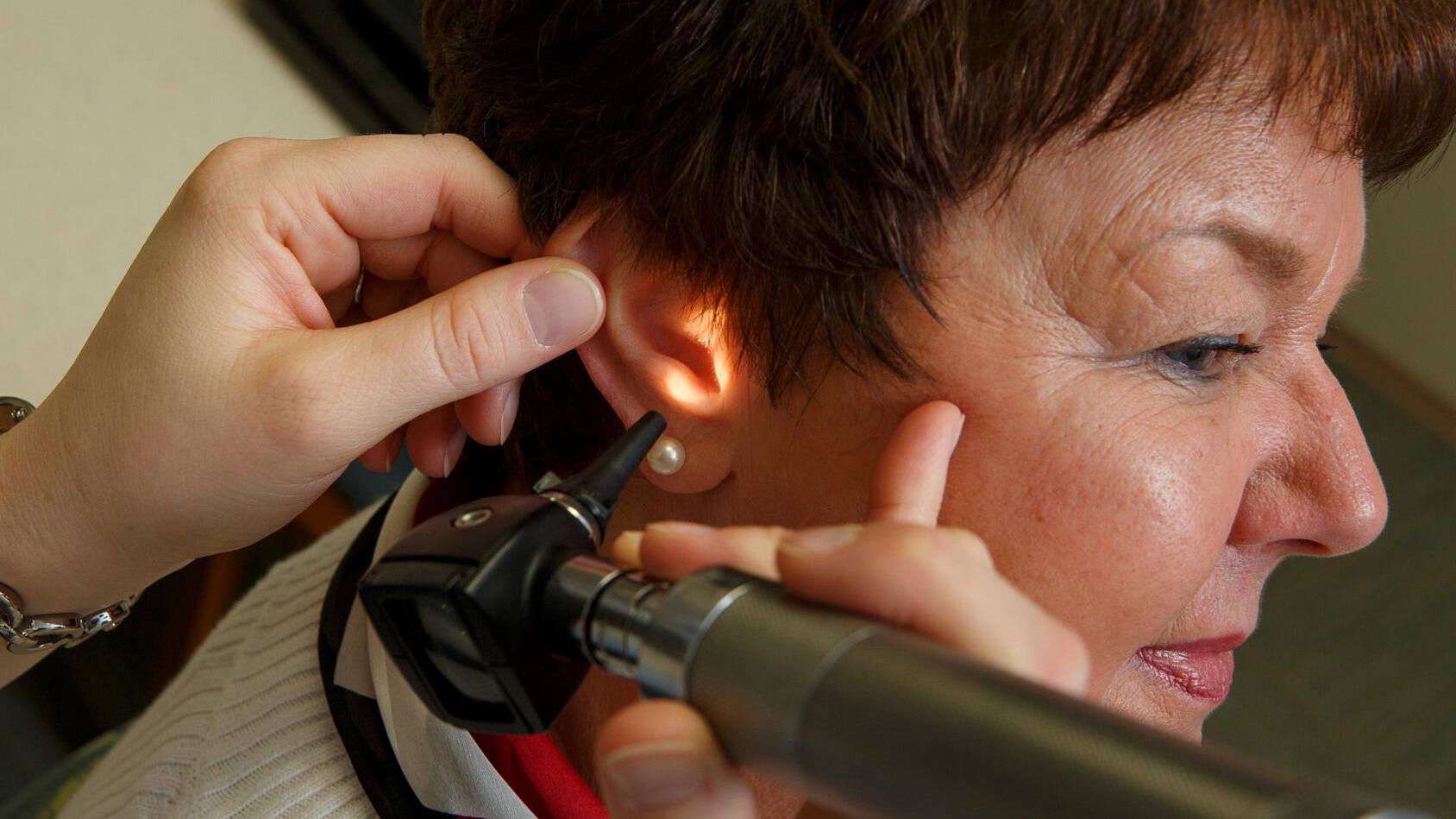This detailed photographic image, set indoors, captures a middle-aged woman undergoing an ear examination. The woman is Caucasian, with short brown hair, lightly adorned with pink eyeshadow, red lipstick, and a pair of white pearl stud earrings positioned at the bottom of her earlobe. She appears calm and slightly bent forward, turning her head from left to right in profile. She is dressed in a white shirt, and potentially wrapped in a beige sweater and a red, black, and white scarf around her neck.

Attending to her is a doctor using an ear scope. The doctor, whose left hand is gently pulling back the woman's ear, holds the ear scope in his right hand. This device features a flashlight, a cone-shaped tip, a magnifying glass, and a handle, designed to examine the ear. In addition to these actions, the doctor's wrist is adorned with a silver bracelet. The image does not contain any text, emphasizing the careful procedure and the serene interaction between the patient and the healthcare provider.